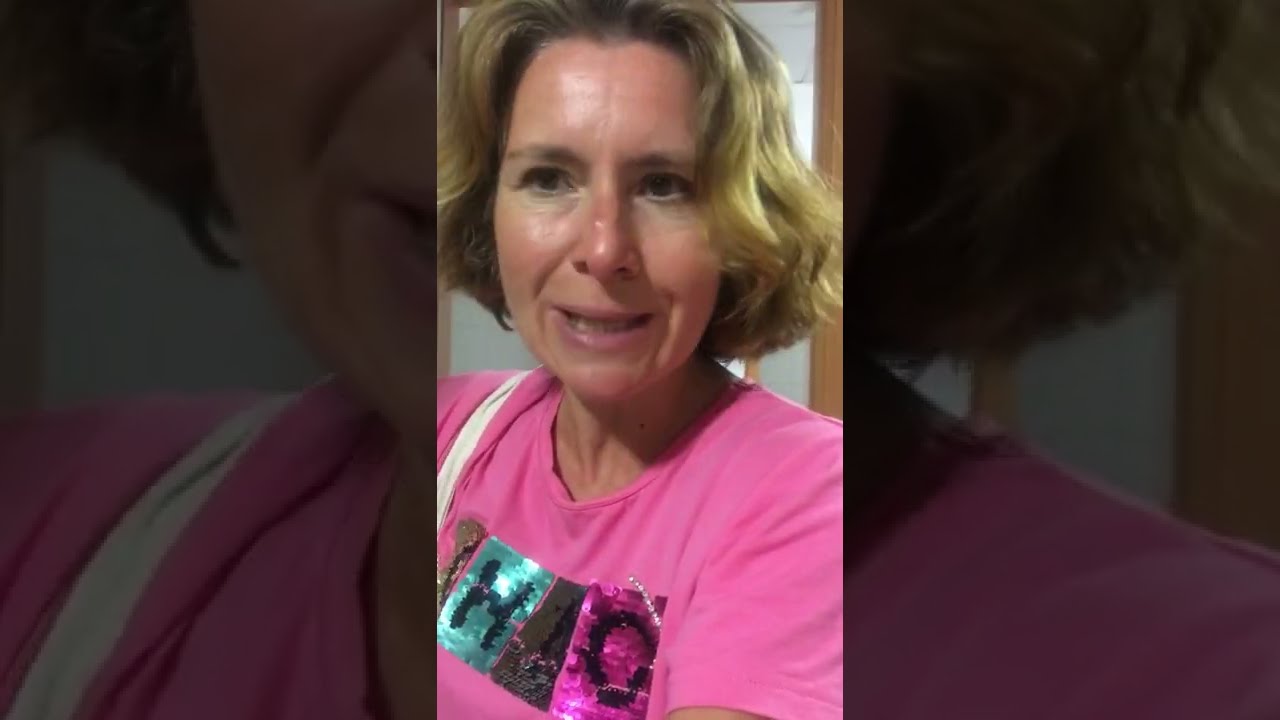This photograph captures a close-up, still shot of a middle-aged woman who appears to be in her late 40s. She has medium-length hair that falls to her chin, with a blend of light brown and blonde highlights. She wears a pink t-shirt adorned with shiny, reflective letters, which seem to be sequined patches forming what looks like an 'H' in a blue patch and an 'O' in a pink patch; the remaining letters are obscured by the crumpled fabric. A beige or white strap from a bag is visible on her left shoulder. Her dark eyes and slightly open mouth suggest she is in the midst of speaking, revealing a bit of her bottom teeth. Her complexion is notably red, and she has a pimple on the left side of her nose. The background hints at an indoor setting, with a doorframe behind her leading to another room characterized by a white ceiling, wall, and light wood trim. The photograph itself is centrally placed within a horizontal rectangle, surrounded by a grayed-out border that mirrors elements of the inner image.